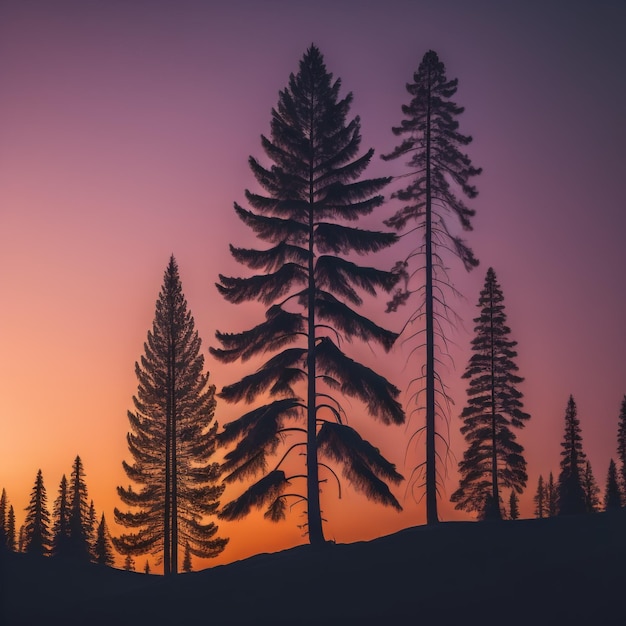This image features an artistic rendering or possibly an AI-generated photo of a striking sunset scene. The sunset sky transitions from deep purples and pinks on the right to lighter orange hues on the left, creating a beautiful gradient effect that darkens towards the top, resembling the onset of night. In the foreground, there are approximately 14 tall pine trees, varying in size and appearance. These trees are silhouetted in a black, monotone shade, offering a captivating contrast against the vivid, colorful sky. Notably, the trees exhibit different characteristics: the one in the forefront has feathery leaves, while others, scattered to the right, display sparsely leafed or barren branches, suggesting they are losing their needles. This combination of vibrant sky and the stark, dark silhouettes of the pines makes for a visually striking and intriguing composition.